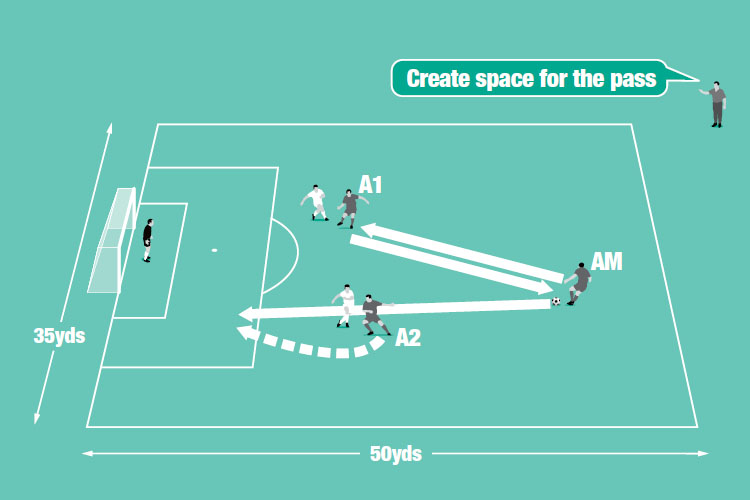The image depicts an instructional diagram designed for illustrating soccer tactics, specifically how to create space for a pass. Set against an aqua-blue background, the diagram showcases a part of a soccer field outlined in white lines, measuring 50 yards horizontally and 35 yards vertically. The depiction includes five players in total: two players in white, three in gray, and a goalie in black. The players are labeled A1, A2, and AM, with AM holding the ball. Arrows illustrate potential passing routes between AM, A1, and A2, showing how to navigate the ball effectively around the field. A speech bubble from an off-field coach emphasizes the instruction, "Create space for the pass," reinforcing the educational nature of the drawing. The entire diagram uses a limited color palette of aqua-blue, teal, black, white, and gray, further emphasizing its illustrative and instructional intent.